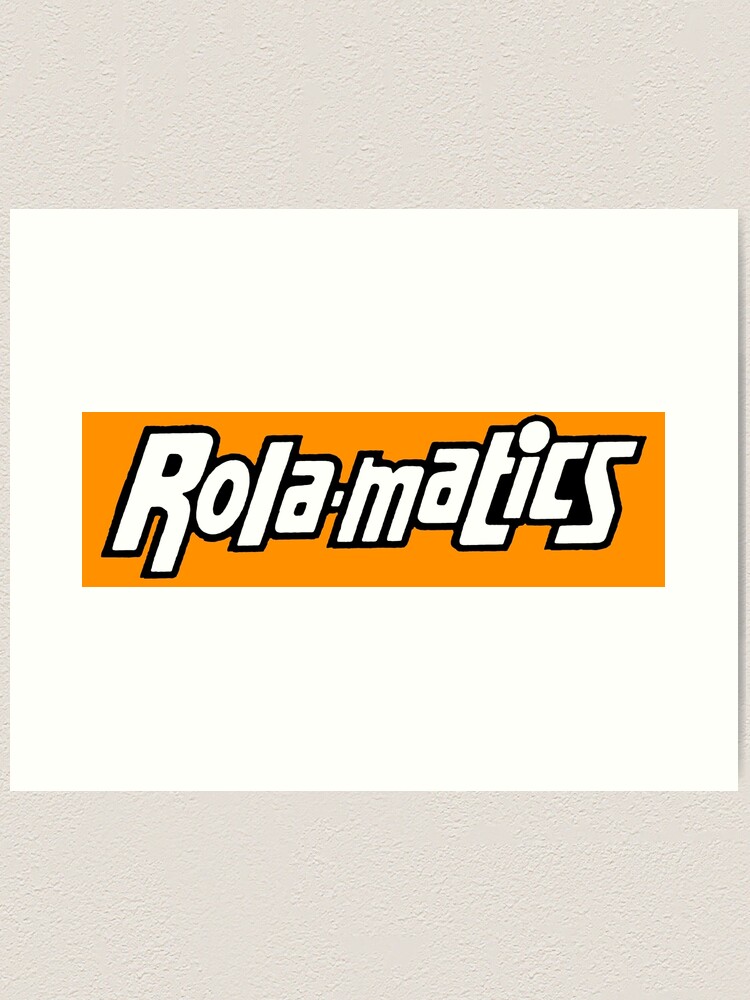The image depicts a gray wall adorned with a large, plain white rectangular canvas. Centrally positioned on the canvas is an orange banner that occupies roughly a quarter of the canvas's space. The banner features the text "Rola-Maddox" in large, white letters outlined in black. The letters are mostly lowercase except for a relatively modestly-sized capital 'R.' Notably, the dot above the 'i' is a larger circle that nearly touches the surrounding 'T' and 'C.' The style of the text is straightforward and clean, contributing to the minimalist look of the overall advertisement, which resembles a long sticker or bumper sticker.